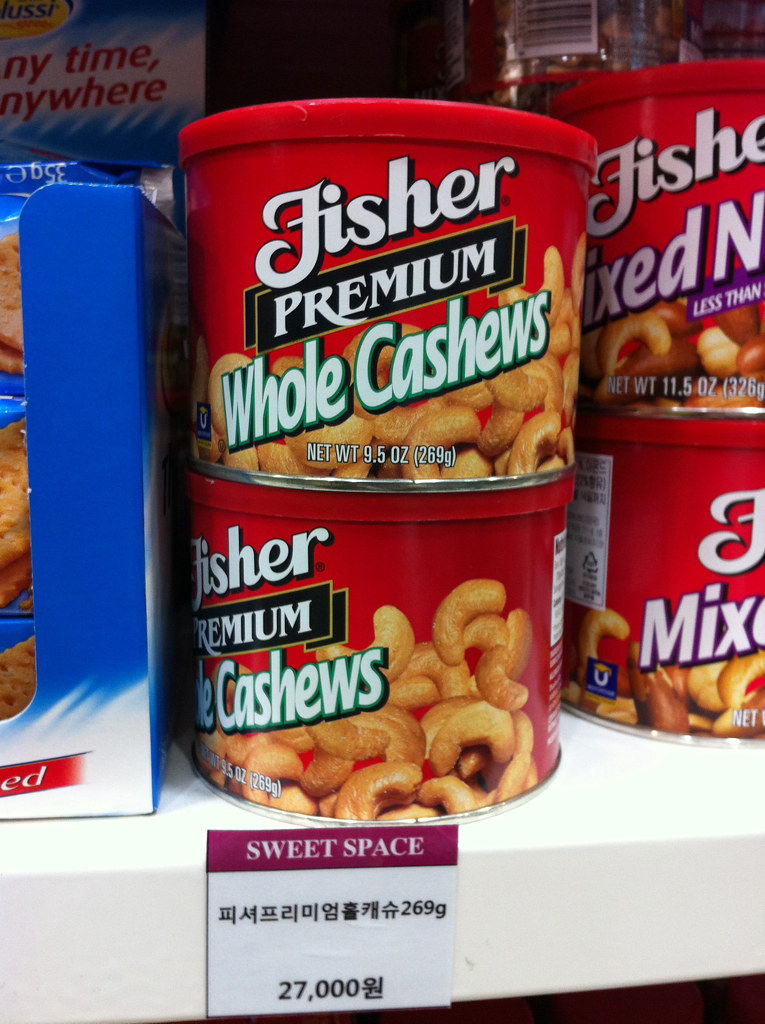A photograph captures a section of a store shelf, which is white in color. A square tag on the shelf features the text "Sweet Space," followed by a series of Asian characters and the number "27,000" accompanied by another Asian character, indicating the price in an unspecified currency. Prominently displayed on the shelf are several red canisters of "Fisher Premium Whole Cashews," marked with the brand name in white lettering. Each canister features an image of cashews. Beside these cashews, more red canisters from the Fisher brand are visible, containing mixed nuts. These cans bear a similar design, showcasing an image of assorted nuts on the label.